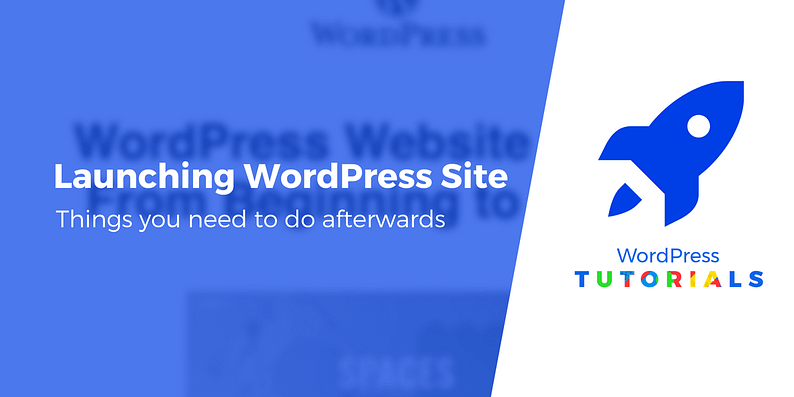In this image, the focus is split into two key sections. 

On the right side, there is a prominent graphic featuring a blue rocket ship, angled towards the top right of the image. Below the rocket ship, the words "Word Press" are written in matching blue text. Following this, the word "Tutorials" is displayed with each letter in a distinct color: the T is blue, the U is green, the next T is blue and red, the O is a blend of blue, red, and green, the R is green and red, the I is yellow and red, the A is yellow and red, and the L and S are both blue. This entire design sits against a crisp white background.

On the left side of the image, a transparent blue overlay serves as the backdrop for white text that reads "Launching WordPress Site. Things you need to do afterwards." Additionally, faintly visible behind this text on the same blue background are the words "WordPress website from beginning to," rendered in black text. Centrally located at the top of the blue section, the word "WordPress" appears along with a small WordPress logo above it.